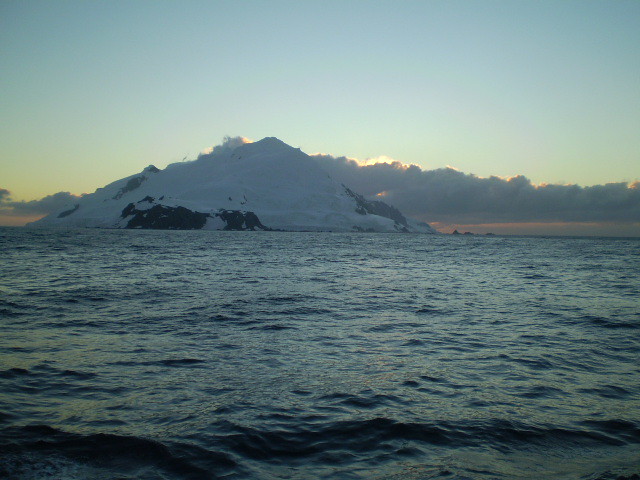Captured from the vantage point of a boat, the image depicts a serene yet striking ocean scene at dusk. The waters exhibit a mix of choppiness and calm, with dark blue, gently rolling waves that suggest recent wind activity or a storm brewing. The ocean stretches towards a majestic snowy mountain, which juts dramatically out of the water, almost appearing as an isolated, snow-capped island. This formidable mountain dominates the background, lightly tinged with reddish hues from the setting sun. The sky above is largely clear, though a line of distant clouds hangs on the horizon. The entire scene is bathed in the subtle, dimming light of evening, with some areas of darkness creating shadowy contrasts on the water. The tranquil yet imposing landscape evokes a sense of cold serenity, possibly suggesting a northern, perhaps Alaskan, location. No signs of human life or other vessels are visible, adding to the pristine and untouched feel of the landscape.